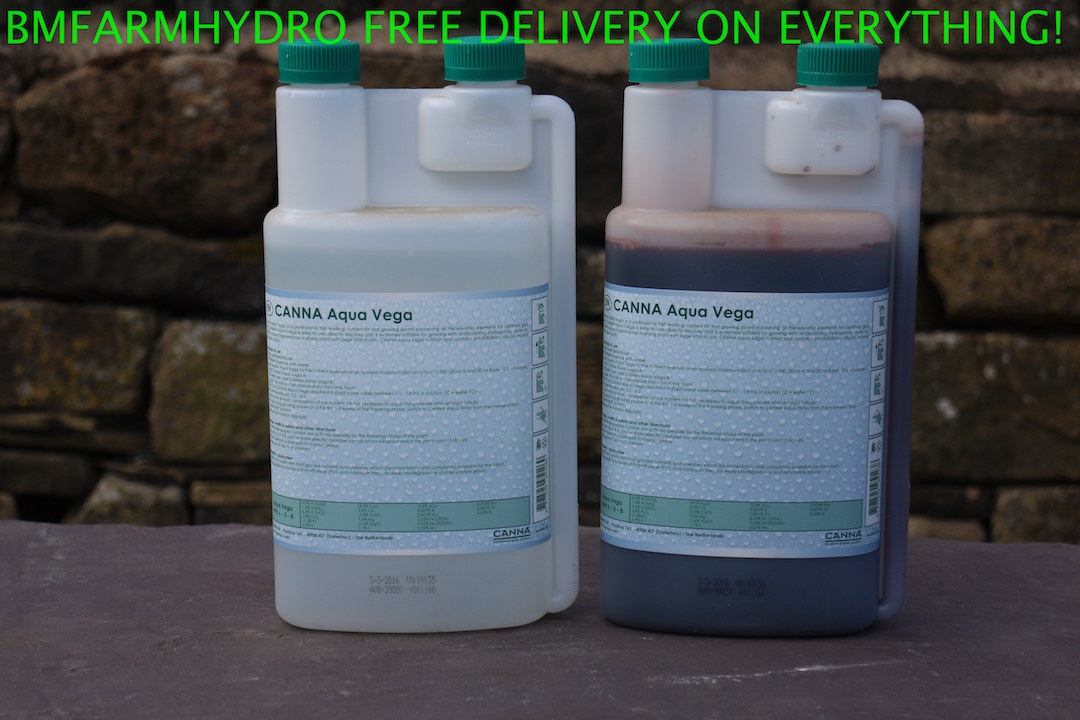The image features two semi-translucent plastic containers with a white hue, each topped with two green caps. The left container holds a clear liquid, while the right one contains a thick, dark red liquid. Both containers are labeled with "Kana Aqua Vega." They rest on a relatively flat stone surface, and the background showcases a stone wall composed of stacked stones. Bright neon green text spans the top of the image, reading, "BM Farm Hydro, free delivery on everything!"